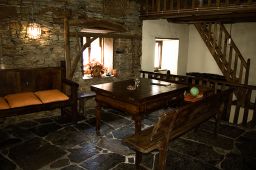This image captures a cozy indoor setting that appears to be a living room or a dining area within a home or cabin. Dominating the right side, a stairwell with a wooden railing suggests stairs going up to another level, with an open door directly beneath. The floor features an intricate stone design, with large black and brown irregular slabs interspersed with white or gray grout. At the center of the room, a square wooden table stands, adorned with various small objects, and bathed in sunlight streaming through a nearby window decorated with flowers. To the left, a wooden seating area or couch is positioned in front of a stone wall, which supports a glowing light fixture hanging above. Additionally, a bench is situated near the table, contributing to the rustic and homely ambiance of this warm and inviting room.